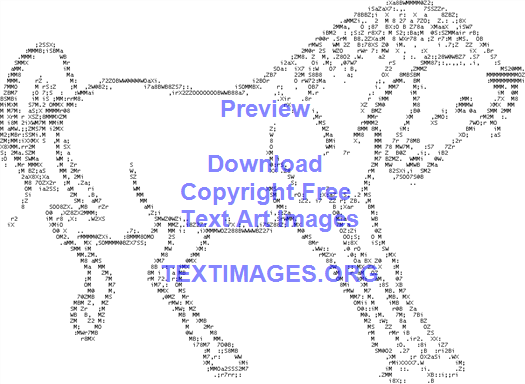This black-and-white image features an intricate line art illustration of a horse, created using an array of tiny black numbers and letters. The horse is portrayed in profile, facing towards the right side of the image with its head bowed forward. One of its back legs is raised in a kicking pose, while its front legs remain straight. The entire horse composition is built from unidentifiable strings of typography, forming the detailed outline and shadowing of the animal. The design is displayed against a white background and spans the full width and height of the image. Superimposed in the center, in purple text, are the words "Preview, download, copyright free text images, textimages.org." This text art captures the essence of graphic design and typography, providing a visually compelling depiction of the horse.